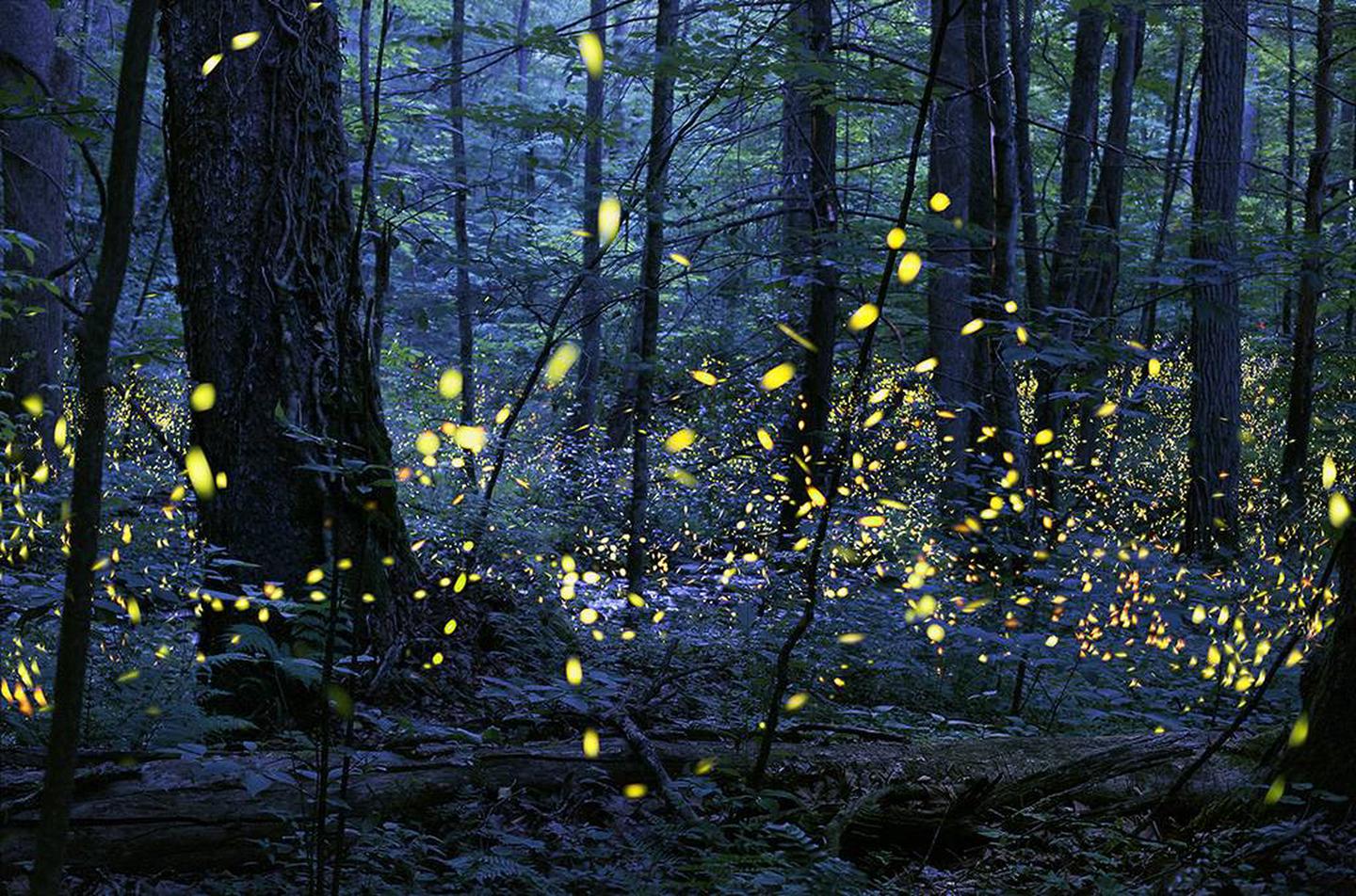This digitally enhanced photograph captures a dense forest scene dominated by a variety of trees. The eye is immediately drawn to an especially large, wide tree trunk on the left side of the image, contrasting sharply against the smaller, stick-like trees that populate the right side and center of the frame. The forest floor is carpeted with leaves, contributing to the earthy feel of the image.

A striking feature of this image is its blue tint, which lends a surreal quality to the scene, making some of the trees appear almost black. Scattered throughout the picture are numerous small, yellow specks that resemble lights. These yellow dots are concentrated mainly in the middle section of the image, creating a visually arresting pattern that appears less dense towards the top and almost absent at the very bottom. Some of these yellow lights look out of focus, suggesting motion, while others in the background appear more defined. The overall effect is one of intricate detail and an ethereal ambiance, as if the forest is illuminated with magical fireflies.